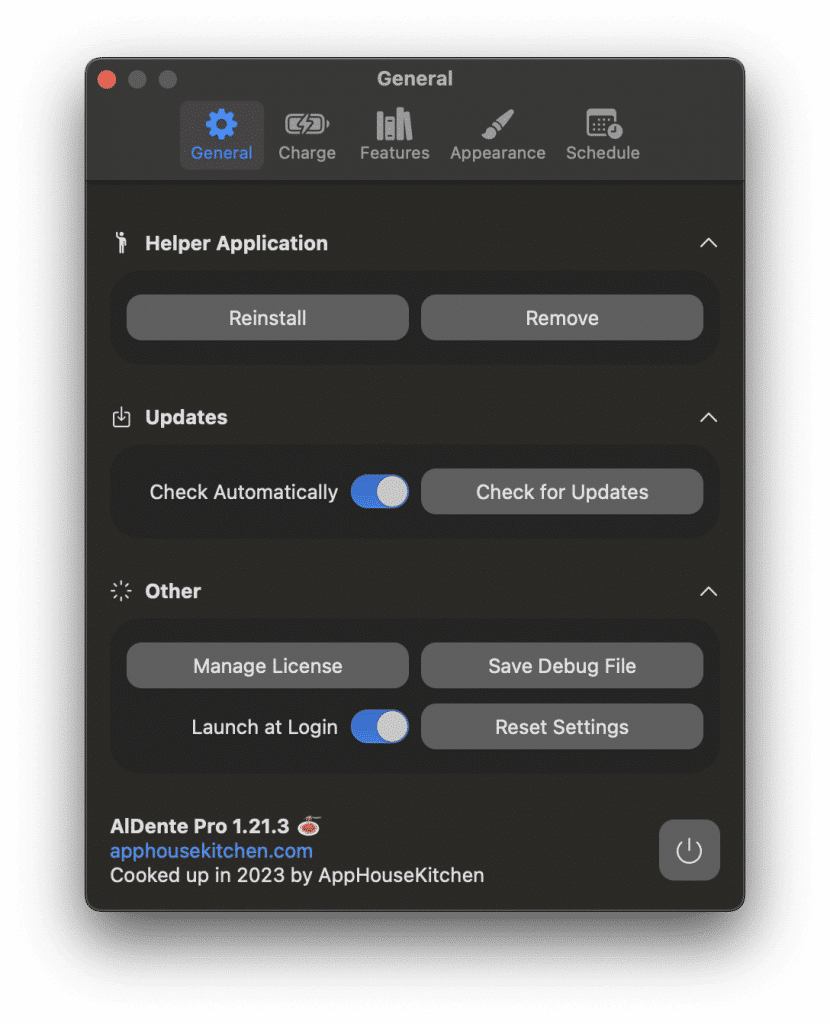This image is a screenshot from a smartphone displaying a dark gray-themed interface. The background color is a very dark gray, with a slightly lighter dark gray border at the very top. On the left side of the screen, there's a navigational menu. At the very top center of this menu, the word "General" is written in gray font. Additionally, "General" appears on the left side in a blue font, accompanied by a circle with notched edges in the same blue color. 

To the right of "General," the word "Charge" is displayed in gray font next to a small image of a battery. Following that, the word "Features" is shown beside a simple schematic of what appears to be four books. Next, "Appearance" is labeled alongside a basic drawing of a paintbrush. Further to the right is the word "Schedule" positioned next to an icon resembling a tiny clock within a black-gray square.

On the right side of the screen, the phrase "Helper Application" is written in white font. Below this are two options, "Reinstall" and "Remove," presented side by side within gray rectangles. Further down, the word "Update" is displayed, followed by a similar setup. Below "Update," the word "Other" is shown, leading to options such as "Manage License," "Save Debug File," "Launch at Login," and "Reset Settings."